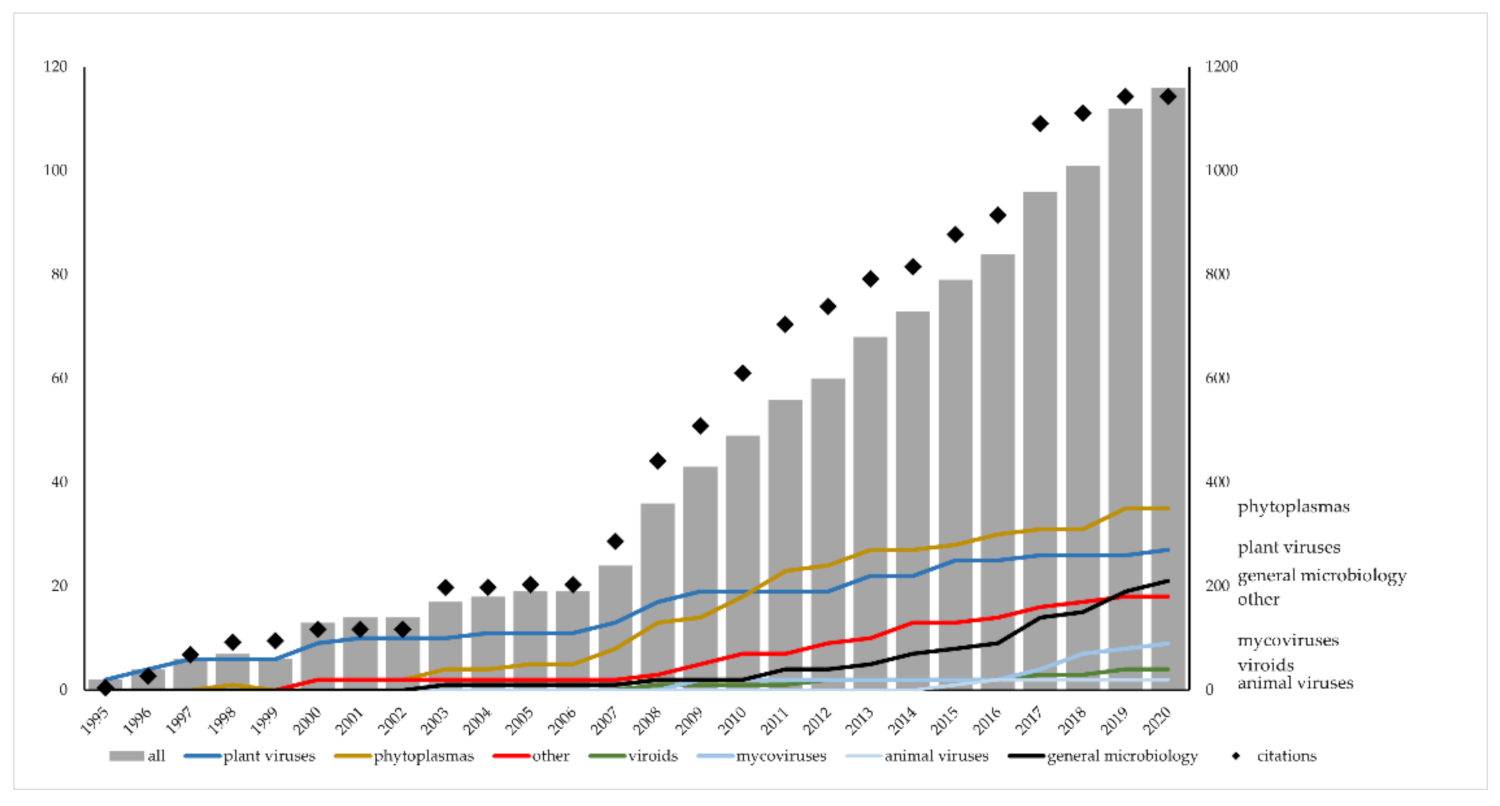The image depicts a detailed bar chart without a title, showcasing data from 1995 to 2021 on the x-axis and has two y-axes: the left y-axis scaling from 0 to 120 and the right y-axis scaling from 0 to 1200. The chart features gray bars progressively increasing in height, alongside a color-coded legend: blue for plant viruses, gold for phytoplasmas, red for other, green for viroids, light blue for microviruses, another blue for animal viruses, and black for general microbiology. Each category is visually demarcated with distinct colors. Additionally, diamond shapes represent citations. The dual y-axis setup offers separate scales, adding complexity to the interpretation of the data.